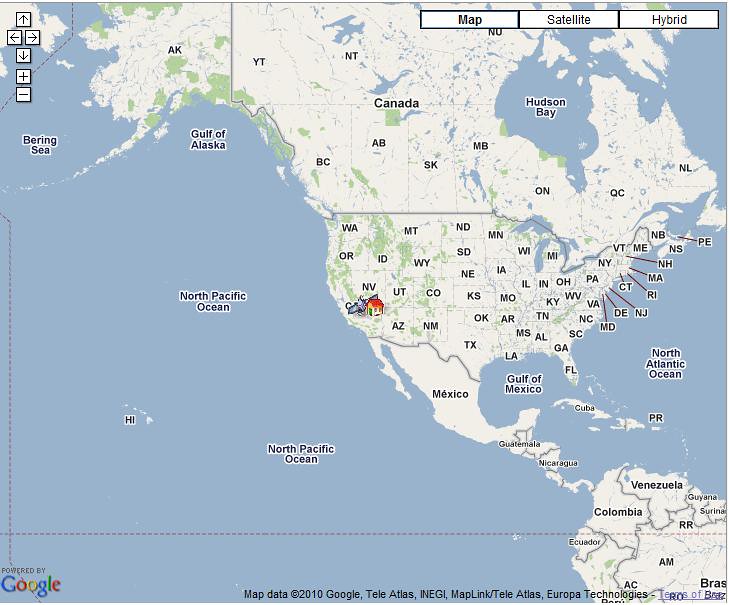This detailed map, primarily showcasing the United States, also includes parts of Canada, Central America, and a portion of South America. The map, provided by Google, uses a predominantly white background for landmasses, accented with green to signify various natural features, possibly mountain ranges. The borders of all U.S. states and Canadian provinces are clearly delineated and labeled with their respective abbreviations. Additionally, Central America is fully displayed, with each country demarcated by borders, while the map extends into South America, terminating around Brazil in the bottom left corner.

Major bodies of water, colored in blue, are also labeled, including the Gulf of Mexico, the Gulf of Alaska, the Bering Strait, and Hudson Bay. The map's interface includes several navigational and informational features: in the top left corner, options for map, satellite, and hybrid views are available, while directional arrows are situated in the top right corner. The Google logo is prominently displayed in the bottom right corner, alongside map data credits to Google, Tele Atlas, and Europa Technologies, dated 2010.

A notable feature on the map is a house icon located roughly in the Nevada area. The house is illustrated with a red roof, white walls, and green doors and windows. Adjacent to the house icon is an indistinct shape that appears to be a satellite or an image of a satellite.